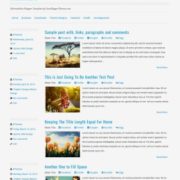**Caption:**

The image features a predominantly gray interface with a layered design. The background is a solid gray color, overlaid by a central gray box containing darker gray text rendered unreadable due to its size. Directly beneath, there are seven clickable gray links that blend with the background.

On the left-hand side of the image, there are 18 or 19 gray buttons vertically aligned, all of which are also unreadable. The right-hand side showcases three notable segments: 

1. At the top, there is larger gray text above a background depicting a striking sunrise or sunset over an African savannah, characterized by tall, spindly trees with foliage at the crown.
  
2. Below, another section reveals more gray text above an image of a lush, green landscape.
  
3. The section beneath that features a clear blue sky with light clouds beneath overlapping trees, framed by additional unreadable gray text.

The limited legibility of the text across the interface, combined with the simplistic and repetitive gray color scheme, dominates the visual narrative of the image.